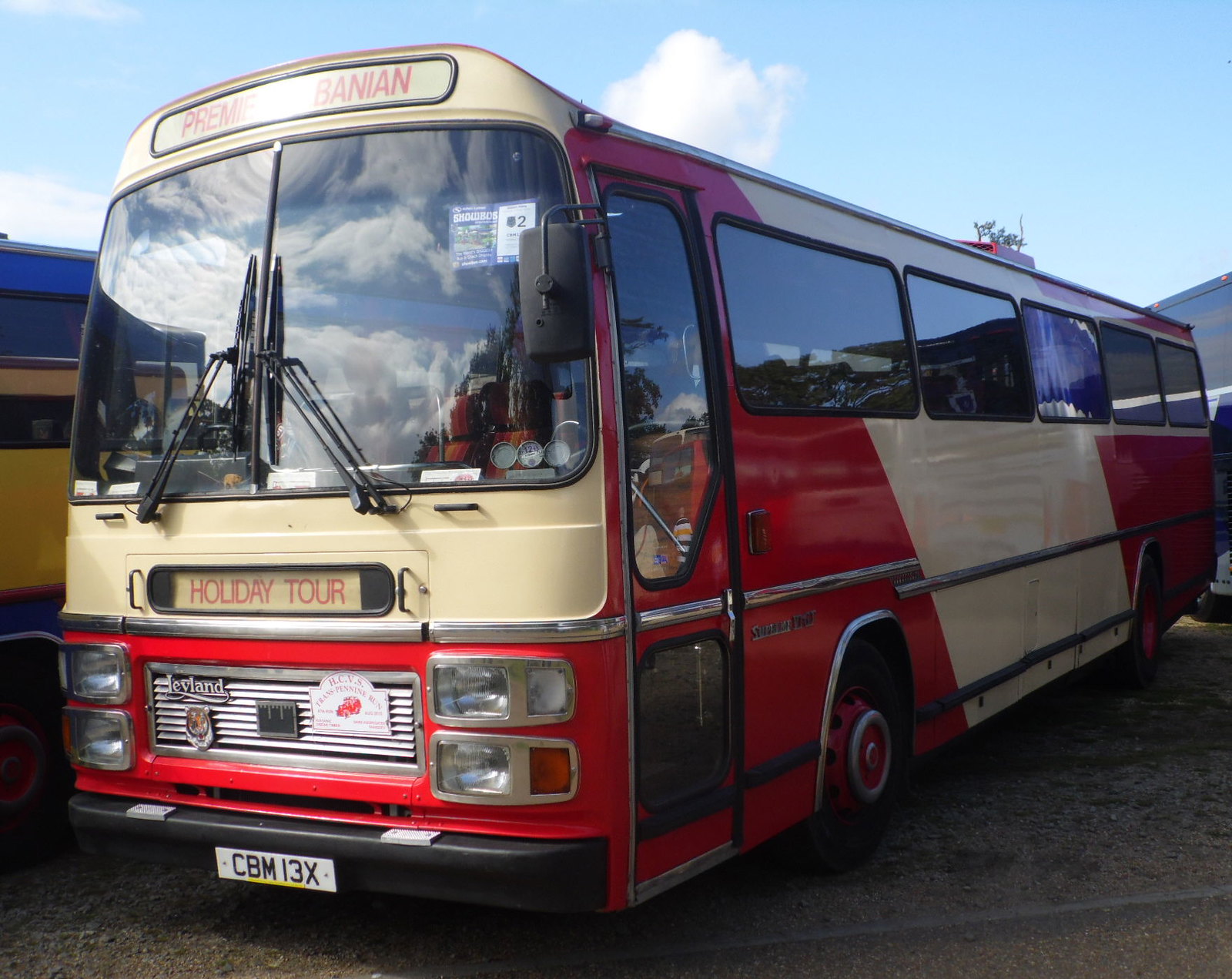The photograph captures a vintage-looking, single-decker tour bus parked on the side of a street under a clear blue sky with a puffy white cloud. The bus prominently features a red and cream paint job with diagonal stripes on the sides and red hubs. The front license plate reads "CBM13X," affixed to a black bumper. Above the large curved windshield, which is divided in the center by windshield wipers, there's a white sign with red writing that likely reads "Premier Banyan," though the R is partially obscured by sunlight. The grille area is marked with "Holiday Tour" in red on a white background. The angled perspective of the photograph allows for a view of the front and the right side of the bus, which has five large windows and a door with two smaller windows. In the background, other buses can be seen, indicating this is possibly a bus terminal or tour starting point. Additionally, a blue and white permit labeled "number two" is visible in one of the windows.